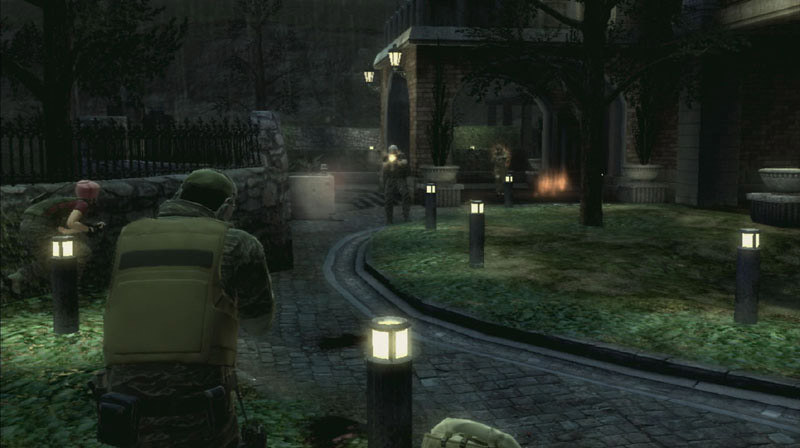This is a highly detailed screenshot from a video game, potentially from a series like Metal Gear Solid or a sniper-themed game. The scene is set during nighttime, adding a layer of tension and stealth to the atmosphere. The location appears to be either a park, a cemetery, or possibly the grounds of an older house. 

The focal point is a cobblestone walkway that begins at the left corner of the image, curving around and extending out of frame, accentuated by evenly spaced black posts with small lights on top, serving as walkway lights. In the right-hand bottom corner stands a man in full military gear: a helmet, a flak jacket, camouflage clothing, and a tactical belt around his waist, all in shades of green. Beside him, to his right, is another man wearing a pink helmet and a red shirt, but otherwise similarly outfitted in green military gear.

A thick stone wall with a black gate lies behind these two men, suggesting a confined or protected area. Within this gated area, a tree stands as a solitary sentinel. The left side of the image shows an expanse of grass, dotted with more of these pedestal walkway lights and a few small trees. 

In the background, there is a stone building featuring archways that form an open portico. Above these archways is a balcony, enclosed by a gate. To the left front of the grassy area, another person dressed in camouflage aims a weapon at the two men in the foreground, identifiable by the flash of light from their gun. This person appears to be wearing a gray helmet. Additionally, another individual is positioned in one of the building's archways, also shooting toward the group in front. More walkway lights are visible in the background, enhancing the scene's eerie and tactical ambiance. 

Overall, the image captures a moment of intense confrontation in a meticulously crafted game environment, evoking a strong sense of strategy and suspense.